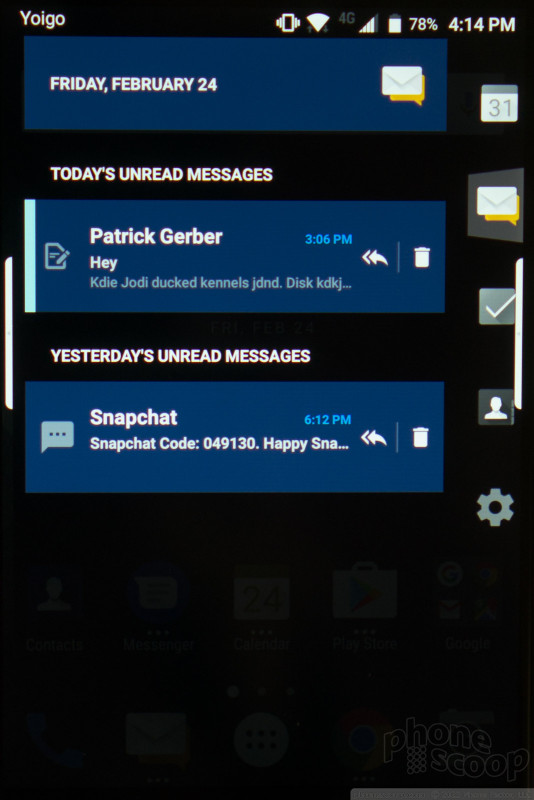The screenshot captures an old mobile phone's display cluttered with various alerts. The wallpaper is largely obscured by the notifications, though faint outlines of app icons are discernible at the bottom. Dominating the top of the screen is a large blue box with the date, "Friday, February 24th," and an envelope icon on the right. Below it, bold white text reads, "Today's Unread Messages," followed by a blue box detailing an email from Patrick Gerber with the subject, "Hey," and a brief snippet of the message in small, light blue font. To the right, it indicates the email was sent at 3:06 PM, alongside reply and trash icons. Further down, "Yesterday's Unread Messages" is prominently displayed, listing notifications from Snapchat about a "Snapchat Code" and an incomplete message starting with "Happy."

A vertical column of icons lines the right side: a calendar page marked '31,' a messages and emails icon highlighted with a light gray border indicating the current selection, an address book icon, and a settings icon. The bottom right corner features a faint watermark reading "Phone Scoop."